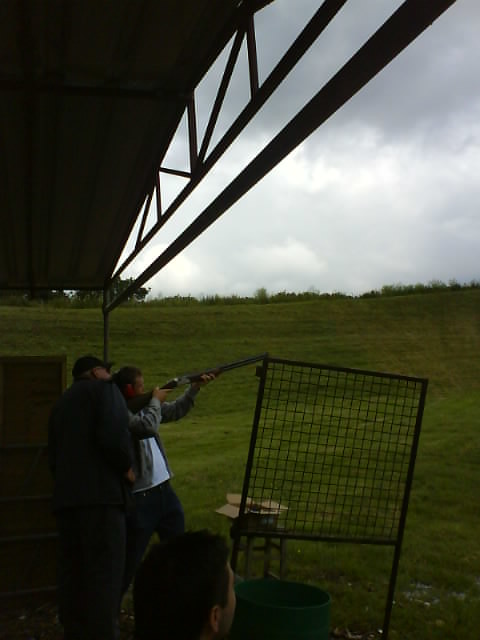In this outdoor image, set in a shooting range, a man is positioned on an incline, aiming what appears to be a shotgun to the right. Standing directly behind him is another man, leaning in to observe the aim. In the foreground and towards the middle, you can see the head of a third man, who is also focused on the direction of the shot. Adjacent to him is a green trash can. To the right of the shooter, there's a metal gate with wire on its upper part, grounded into the dirt. The scene is framed by a sprawling green field that extends to the horizon, featuring bushes, tall grasses, and trees. A constructed awning with a metal frame covers the men, offering shade, and portions of the blue and white cloudy sky are visible through the structure.